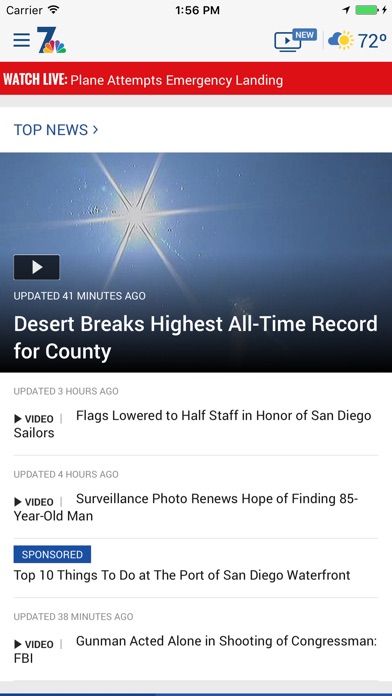The image depicts a web page displayed on a cell phone screen. The following elements are visible:

1. At the top, the status bar shows:
   - "1:56 p.m."
   - The phone carrier labeled as "Carrier."
2. The main page features:
   - A temperature reading of "72 degrees" in blue on the right side.
   - A green battery icon indicating the phone's battery level.
   - A blue box labeled "New" with an arrow.
   - An icon showing a cloud with sunshine.
   - An image of a "7" symbol, resembling the colorful NBC peacock logo, likely indicating a network or channel.
3. A red strip banner runs across the top part of the page with the headline: "Watch live: Plane attempts emergency landing."
4. Below the banner, there is a section titled "Top News" in blue.
5. A large clickable video thumbnail is featured with the headline: "Desert breaks highest all-time record for County," marked as "Updated 41 minutes ago."
6. Additional news segments include:
   - "Video of sailors."
   - "Video of 85-year-old man: Hope of surveillance photo renews hope of finding him."
   - A sponsored article titled "Top 10 things to do at the Port of San Diego waterfront," noted as "Updated 38 minutes ago."
   - "Video: FBI gunman acted alone in shooting of congressmen."

The layout is informative, blending news updates with visual content and sponsored articles.